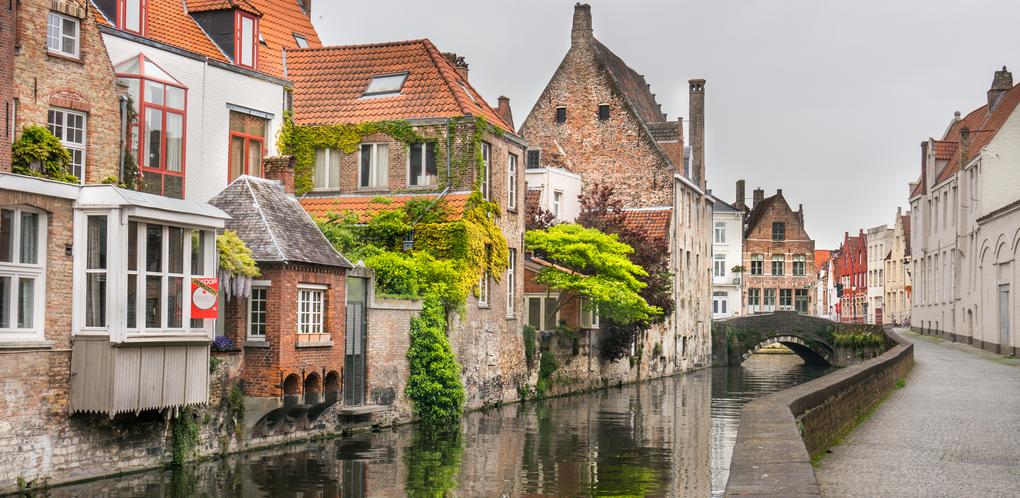The image depicts a quaint European town, reminiscent of Venice, with a winding canal that starts at the bottom left corner and meanders upwards to the right, before continuing straight. Flanked by ancient, weathered buildings built from red brick, stone, and grayish materials, the canal is about 40 feet wide. The left side showcases contiguous structures, with some featuring second-level windows that jut out and others adorned with greenery and vines that cascade down to the water. Spanning the canal is a dark gray stone bridge, adding to the medieval ambiance.

Along the right side of the canal, a short stone wall with a ledge is adjacent to a pathway constructed of gray brick pavers, which eventually leads out of the image at the bottom right corner. This pathway is bordered by buildings that begin around the middle of the image and continue to the left, including light-colored facades and one notable red building further down the street. The buildings on this side feature variations of white and red-framed windows, some Cape Cod style, and steeply pitched roofs with chimneys.

Throughout the scene, there are patches of greenery, including tops of green and red trees interspersed between the buildings. Overhead, a light gray sky looms above, with dark clouds hinting at an overcast day. All these elements combine to create a picturesque, almost medieval town scene, likely somewhere in Europe, steeped in history and charm.